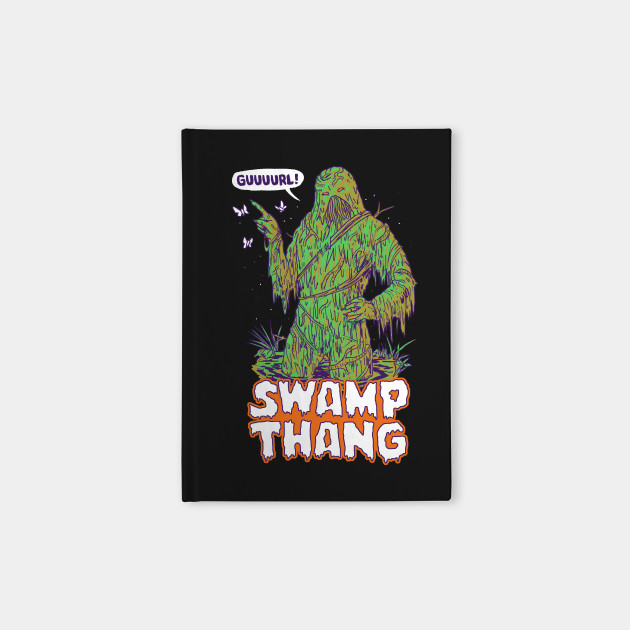In the center of the image, perfectly aligned against a serene gray background, is a vertical, rectangular poster or possibly a magnet designed in a cartoonish and humorous style. The poster's background is entirely black, drawing immediate attention to the vibrant and detailed artwork. Dominating the scene is a swamp creature, humorously titled "Swamp Thing." The creature, depicted in various shades of green and yellow with blue accents, stands upright from the thighs up. It has one hand on its hip and the other pointing upwards. Surrounding it, there's green and yellow water with patches of grass and a few butterflies or bugs flying near its extended finger. Two pieces of text are prominently featured: a blue exclamation bubble at the top exclaims "GUUURL!" with vibrant, playful letters, while the bottom text, "SWAMP THANG," is written in white and encased in an orange, dripping design. The colors in the image are diverse, including green, brown, white, beige, black, orange, and purple, all contributing to the lively and humorous tone of the artwork.